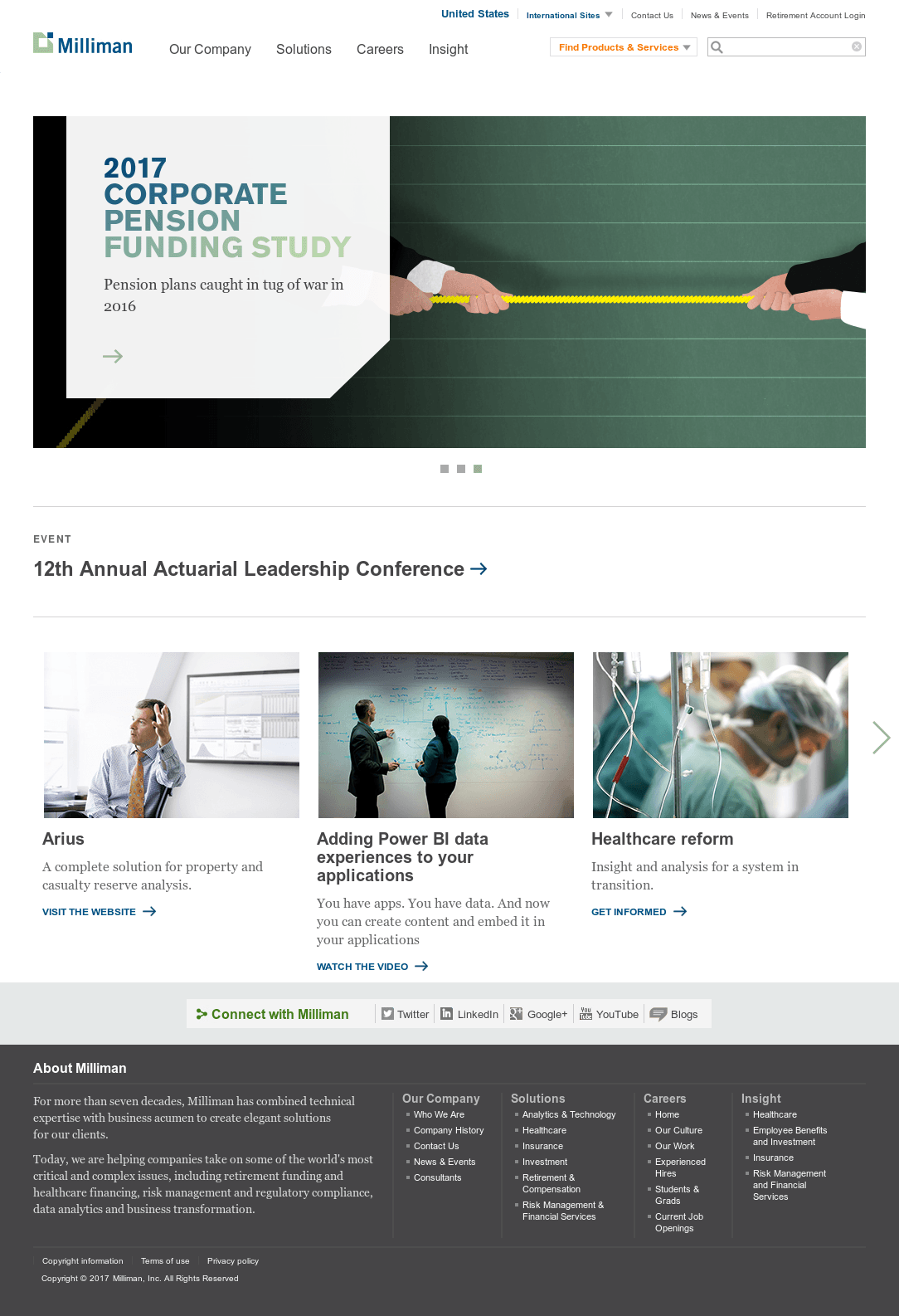This webpage layout for Mealyman is characterized by a variety of navigation options and informative links. The top navigation menu contains sections for "Our Company," "Solutions," "Careers," "Insights," "United States," "International Sites," "Contact Us," and "News and Events." 

A prominent banner highlights key offerings such as the "2017 Corporate Pension Funding Study" and an article titled "Pension Plans Caught in Tug of War in 2016." There are also announcements about upcoming events, including the "12th Annual Actuarial Leadership Conference."

To the right of these sections is a search field, facilitating easy access to the website’s content. Beneath the banner, detailed descriptions of specific solutions are provided, such as "A Complete Solution for Property and Casualty Reserve Analysis" and an invitation to "Visit the Website."

The site also advertises the integration of bi-data experiences into applications, encouraging users to "Watch the Video" to learn more. Health care reform insights and analyses are available for those looking to get informed about this transitioning system.

At the bottom of the page, Mealyman makes it easy to connect via social media platforms including Twitter, LinkedIn, Google+, YouTube, and various blogs. There's also an "Account Login" area and options to "Find Products and Services."